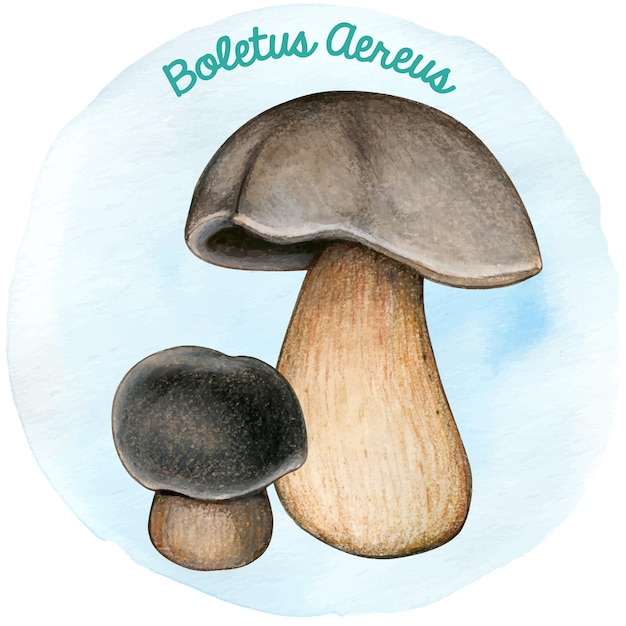The image depicts two mushrooms rendered in a combination of colored pencil and watercolor. Set against a light blue circular background with dark blue splotches, the smaller mushroom on the left stands at half the height of the larger one on the right. The left mushroom features a rounded black cap and a stem that fades from light to dark brown. The larger mushroom on the right showcases a tall stem, a somewhat less round, half-sphere cap predominantly brown with hints of black, and a shadowed interior. Above the mushrooms, in a sea green, curving cursive font, the title "Boletus Aereus" is inscribed.